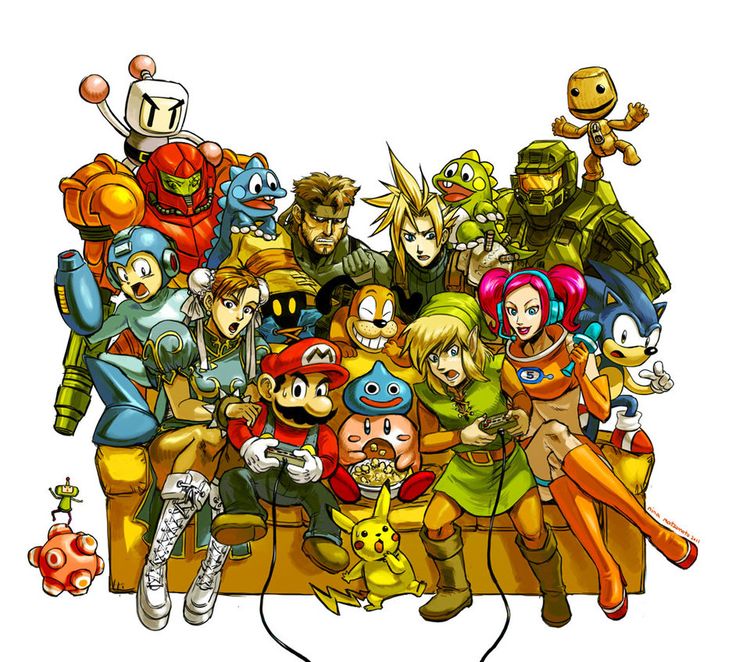The image is a highly detailed, hand-drawn artwork that features a diverse ensemble of iconic video game characters gathered around a yellow couch set against a white background. At the center of the floor, Pikachu sits with a surprised expression. Above him, Kirby is perched on the couch, with a Slime from Dragon Quest atop Kirby. On the couch, from left to right, are Mario holding a video controller, Chun-Li from Street Fighter, Link from The Legend of Zelda, Ulala from Space Channel 5, and Sonic the Hedgehog. Mega Man and Ulala flank the edges of the couch.

Standing behind the couch and leaning over are even more characters: Bomberman clings to Samus Aran in her iconic suit, a dragon from the Bubble Bobble series sits upon a Black Mage from Final Fantasy IX, Solid Snake from Metal Gear Solid is observed next to Cloud Strife from Final Fantasy VII, who stands beside another Bubble Bobble dragon. Master Chief from Halo stands sturdily with Sackboy from LittleBigPlanet on his shoulder. Additionally, to the far left next to the couch, the Prince from Katamari Damacy is positioned rolling a Katamari ball, adorned with many sphere-like bumps. The entire scene captures a nostalgic and vibrant celebration of video game lore.